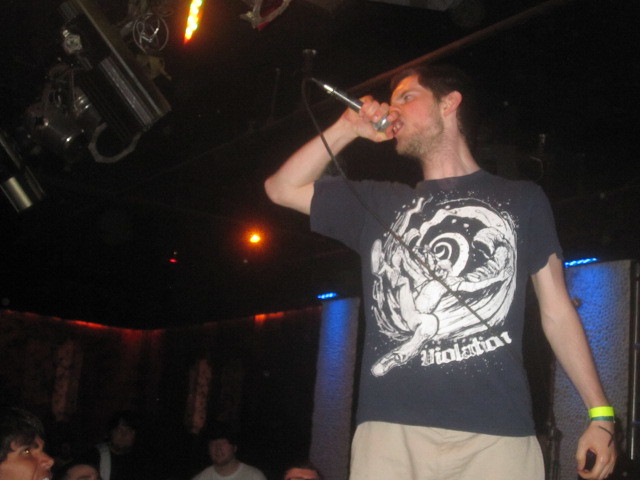In this nighttime indoor photograph, a man is captured singing passionately on stage at what appears to be a concert venue or bar. The scene is dimly lit, with no bright stage lights turned on, creating a somewhat blurry image, though the central figure remains identifiable. The singer, standing at the center of the image, wears a short-sleeved black t-shirt with a graphic of a person falling into a vortex, labeled "Volition." On his right wrist, he has a yellow and blue bracelet—likely an entry band for the venue—and another possible gray wristband or watch, with an X marked on the back of his hand in black ink. He also sports khaki shorts or pants and has short brown hair. The microphone is held close to his mouth, almost muffling his singing, with its cord visible trailing around his body. In the background, audience members are seen looking up towards the stage, adding to the intimate atmosphere of the performance.